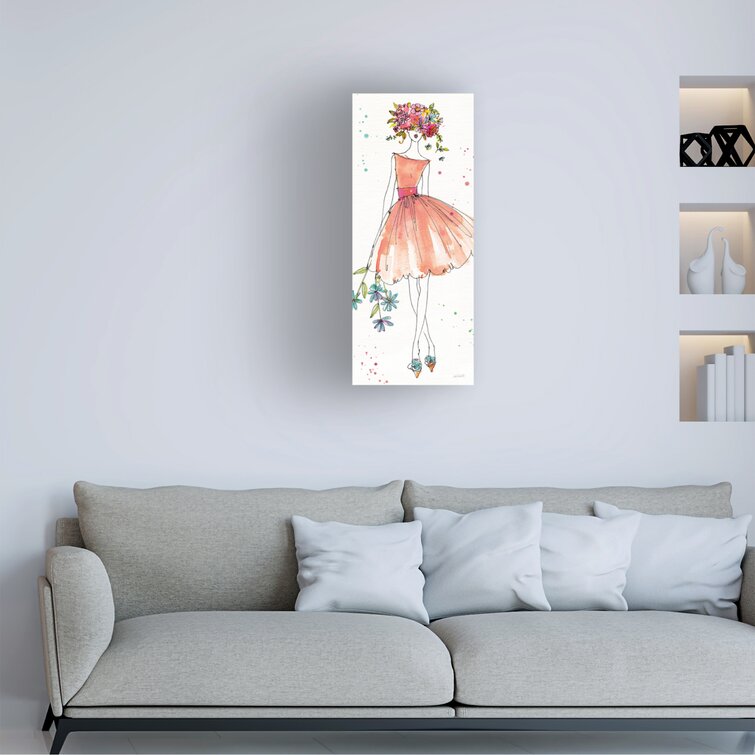In this detailed photograph of a modern living room, a low-sitting gray couch with short legs dominates the lower part of the image. Positioned centrally on the couch are four small, silvery white throw pillows arranged to the right. The wall behind the couch is a light cream or gray hue, lending a calm ambiance to the space.

Mounted prominently on the wall is a long rectangular canvas featuring a hand-drawn image of a woman. She wears a striking peach-colored, ballerina-like dress, accentuated with a red waistband. Holding flowers in varying shades of blue and turquoise in her right hand, her head is adorned with a lavish bouquet of pink, yellow, and purple flowers, merging traditional portraiture with floral exuberance. Decorative dots in blue, red, and orange embellish the white background, adding an artistic touch. The woman’s face is slightly out of focus, but her reddish-purple lips are distinctly visible.

To the top right above the couch, three open alcoves are integrated into the wall, each displaying unique decorative items. These niches contain out-of-focus white books, elegant swan statues, and hexagonal structures, contributing to the room's sophisticated aesthetic. The shelves further complement the room with their subtle white background, seamlessly blending into the overall décor.